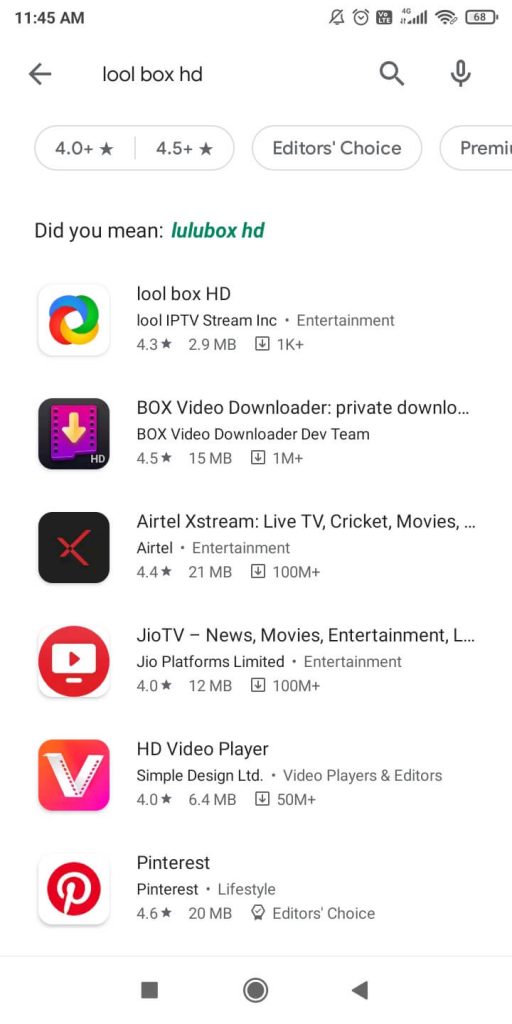A screenshot taken on a mobile phone displays a Google search page at 11:45 a.m. with the battery level at 6%. The search query entered is "Lulebox HD". The Google search suggestions feature prominently, including "Lulebox HD," "box visual downloader," "private download," and apps like "Airtel Xtreme," which is highlighted as "Xtreme," Live TV apps, cricket apps, "Geo TV," news apps, movie apps, and entertainment apps. There's also an HD Video Player by Simple Design Limited and Pinterest at the bottom of the visible suggestions. The background is white, with each suggestive thumbnail showcasing their respective app logos, characterized by a range of pinks, reds, and purples, adding vibrant hues to the interface.